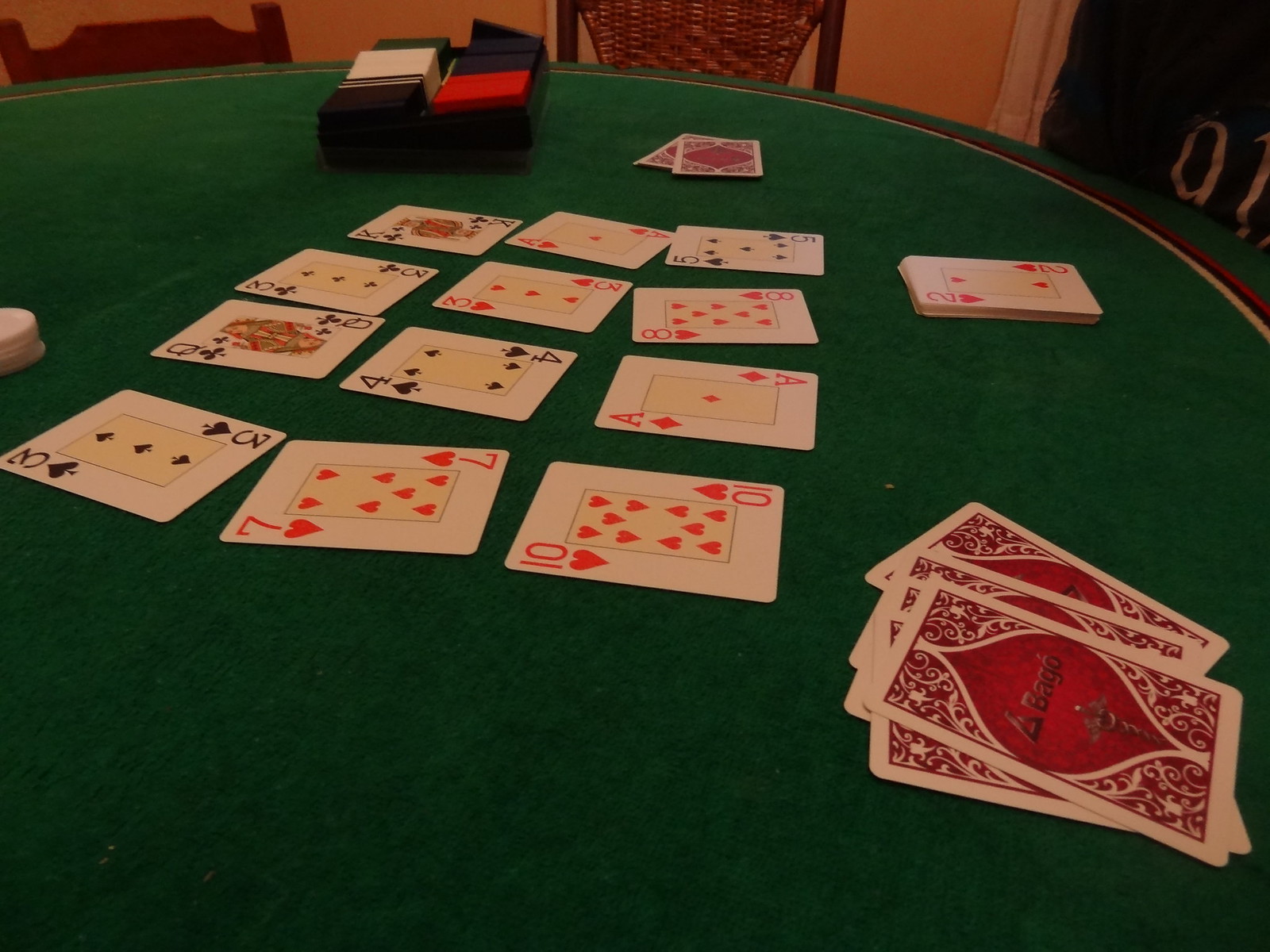The image features a round card table covered in green felt, quintessentially designed for card games. Dominating the scene, the table occupies approximately 90% of the photo, with the focus directed towards the assortment of playing cards and the card dealing machine placed slightly off-center at the top right. This sleek, black machine contains a white deck on its right and a red deck on its left.

Around the table, in the top right corner and top center, the backs of two chairs are visible. The chair on the right has a wooden back, distinguished by its visible grooves, while the center chair exhibits a wicker middle framed by brown slats. To the left of these chairs, the yellowish color of the wall adds a warm backdrop to the setting.

On the table, three rows of face-up cards are meticulously laid out, progressing from closest to the camera to the furthest:
- The first row features the Three of Spades, Queen of Clubs, Three of Clubs, and King of Clubs.
- The second row displays the Seven of Hearts, Four of Spades, Three of Hearts, and Ace of Hearts.
- The third row comprises the Ten of Hearts, Ace of Diamonds, Eight of Hearts, and Five of Spades. 

Beyond these, two cards lie face down, suggesting an element of suspense or ongoing gameplay. Below this arrangement, a small stack of cards is topped by a face-up Two of Hearts. Closer to the bottom left of the image, four face-down cards are arranged, each adorned with a pattern of red spades against the traditional card background.

This detailed composition provides an immersive glimpse into a moment frozen in a card game, rich with textures and subtle details.